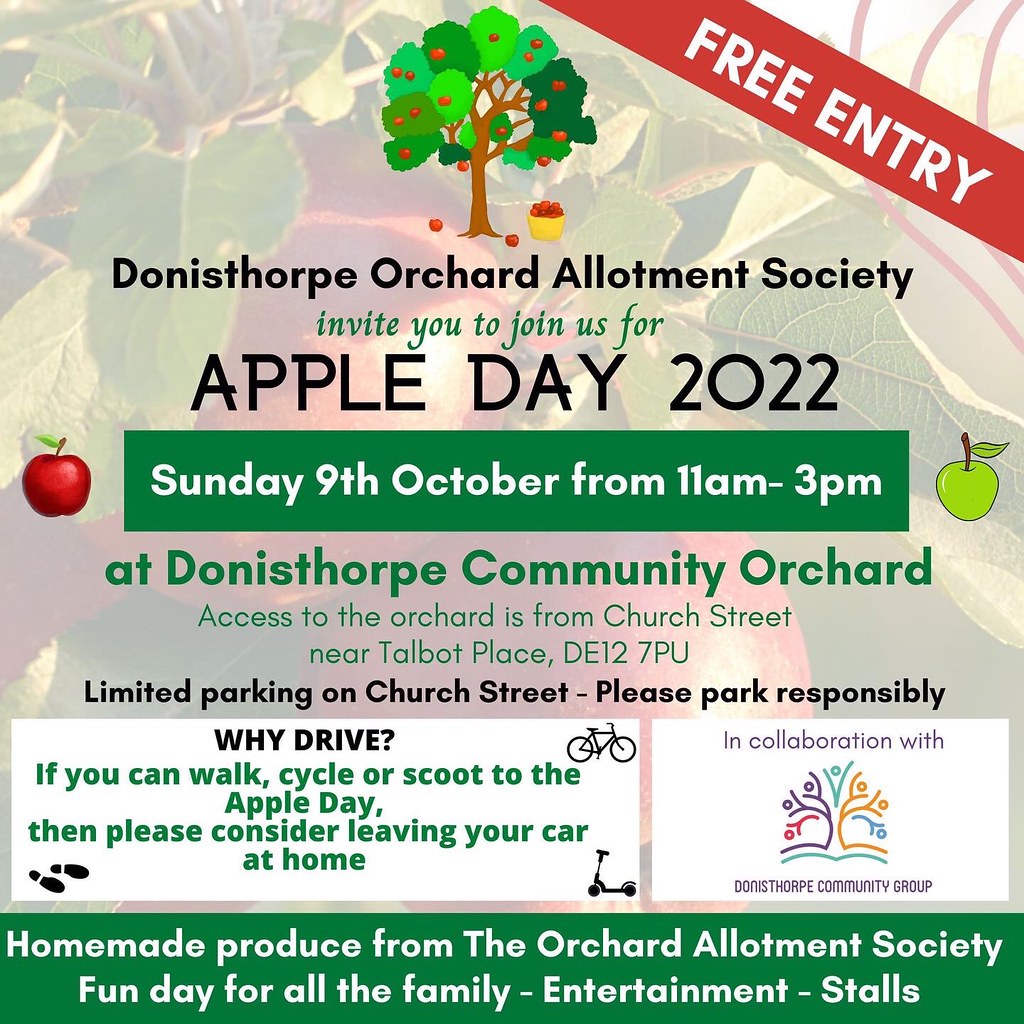The advertising flyer for "Apple Day 2022" is richly designed with a vibrant background featuring a close-up photograph of several apples growing on a tree amidst lush green leaves. A prominent red banner with white text that reads "FREE ENTRY" runs from the top middle to the upper part of the right side of the image. Centrally located at the top is a charming cartoon graphic of a tree laden with red apples, complemented by a yellow basket filled with apples at its base. Beneath this illustration, in black text, is the name "Donasthorpe Orchard Allotment Society," followed by green text inviting viewers to "join us for" the event. Central to the flyer is a large, bold announcement in black text that declares, "Apple Day 2022."

Further down, between a red apple on the left and a green apple on the right, a green bar with white text provides the event details: "Sunday, 9th October from 11 a.m. to 3 p.m." Additional text in green specifies the location: "at Donsethorpe Unit Community Orchard," with directions explaining that access is from Church Street near Talbot Place. A note in black text advises about limited parking on Church Street, urging attendees to "park responsibly."

In the bottom right corner, a colorful icon announces the collaboration with the "Donasthorpe Community Group." On the left-hand side, the flyer suggests sustainable travel options with images of a bike, scooter, and footprints, encouraging visitors to leave their cars at home. The bottom section highlights additional attractions, noting "homemade produce from the Orchard Allotment Society," "fun day for all the family," and entertainment with stalls.

This beautifully detailed and informative flyer effectively mixes real imagery with graphics and colored text to create an inviting and engaging advertisement for a community event.